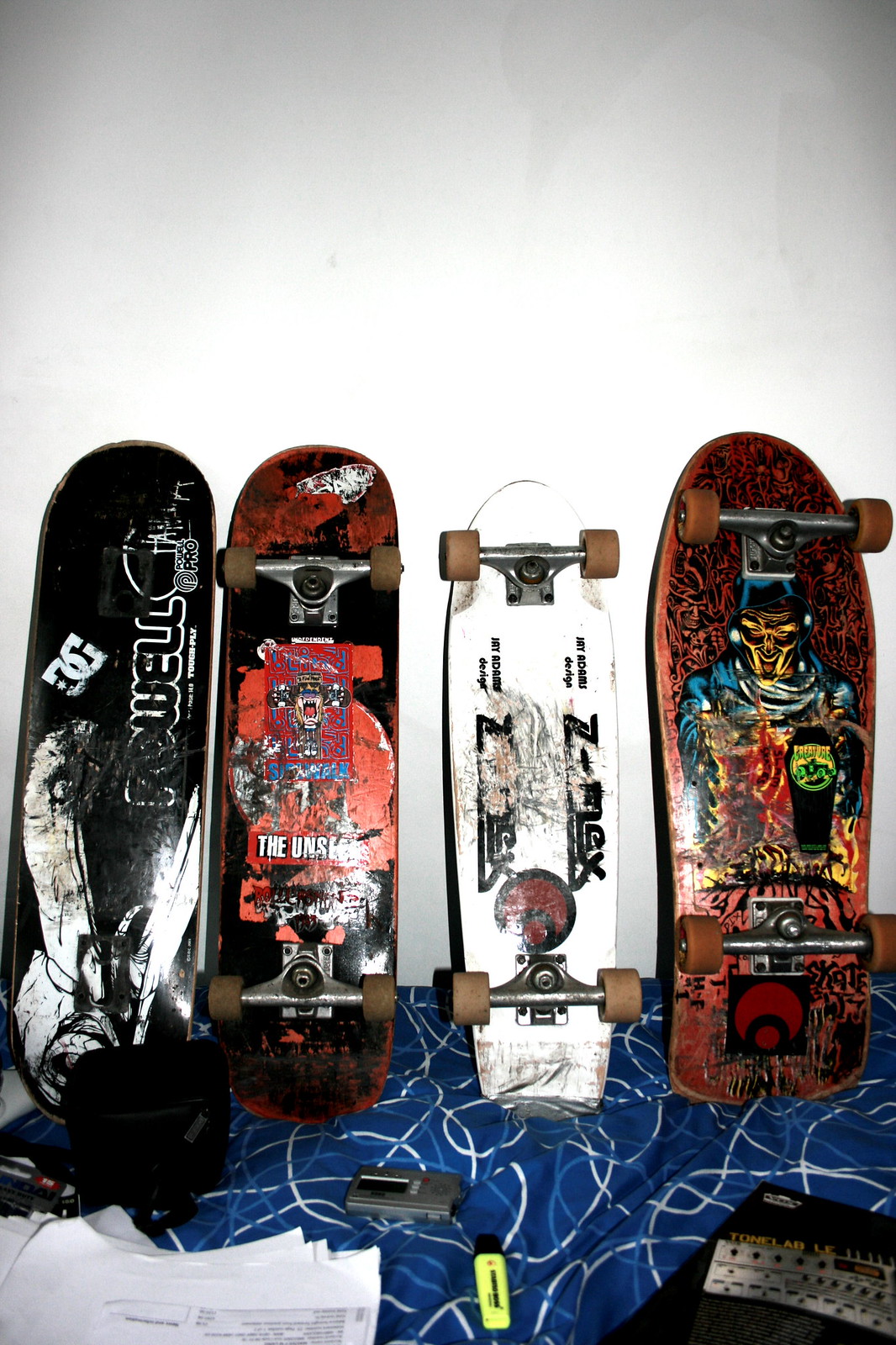This detailed image showcases four distinctive skateboards leaning against a white wall, each positioned on top of a dark blue comforter adorned with lighter blue and white patterns of circles and swirls. The skateboard closest to the left is primarily black with some white highlights and appears to have "DG" emblazoned on it, though some of the lettering is worn and hard to read. Next to it is a red and black skateboard featuring a sticker that says "The Unseen," with red wheels adding to its striking appearance. The white skateboard in the center is marked by black writing and a red emblem, though the writing is partially scuffed and unclear. The fourth skateboard to the right is orange with a black geometric pattern and showcases a yellow skeleton wearing blue clothing, accompanied by red wheels. Surrounding the skateboards, the comforter hosts various items, including a pile of papers, what looks like a highlighter, possibly a cassette recorder, a lighter, a t-shirt, and items that are too obscure to identify. This vivid array forms a colorful and textured scene, emphasizing the unique character of each skateboard and the miscellany of objects resting on the bed.